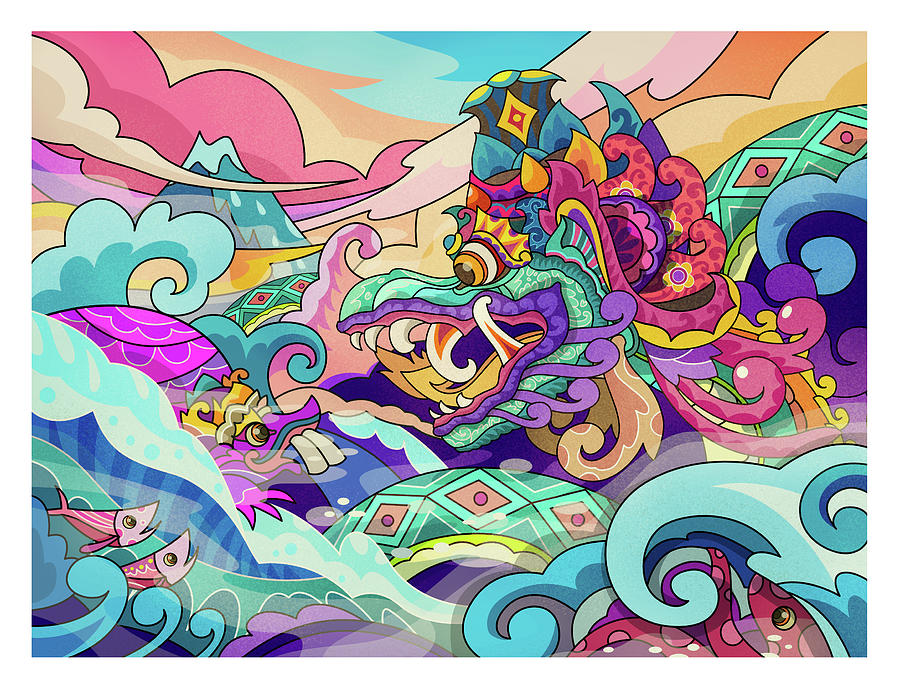This vivid, psychedelic image appears as a colorful, surreal, and detailed digital artwork, potentially resembling a cartoon or animated piece. The square canvas, devoid of a border, background, text, or artist's signature, features an extraordinary dragon bursting from the lower right-hand corner toward the center. Its head, an eclectic mix of purples, yellows, greens, and blues, is adorned with a three-pointed feather-like crown, teal-rimmed with a yellow diamond center, boasting a smaller red diamond within, and an observable eye. The dragon's mouth is open wide, revealing massive, long, curled teeth and a peculiar flame-shaped tongue. Surrounding it, various aquatic elements, including a couple of fish and an octopus in the lower left, hint at an underwater setting. The upper left corner showcases a mountain with a backdrop of swirling clouds colored in white, purple, pink, yellow, and blue. The scene is filled with black shapes adding to the artistic, cartoonish, and trippy atmosphere, with the primary hues being blue, beige, pink, and muted greens. This intricate design could serve as both a striking poster and a detailed artistic exploration.